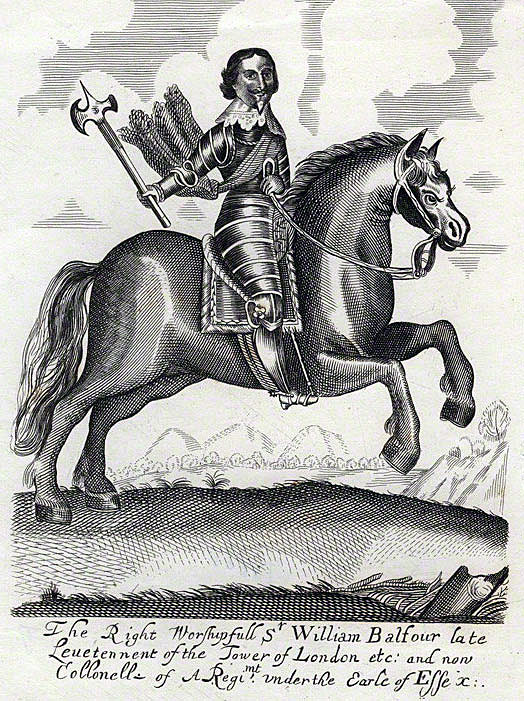The black-and-white old-style illustration, done in an early 1800s block print style, features a detailed depiction of a man riding a rearing horse. The man, identified as William Balfour, late lieutenant of the Tower of London and now a colonel under the Earl of Essex, is clad in armor with a lacy, frilly collar and a sash across his shoulder. He has short, dark hair and a pointed goatee. In his right hand, he brandishes a sharp, spiky axe, while his left hand grips the horse's reins. The muscular horse, shown in an action pose with its front legs off the ground, gallops across an etched grass landscape. The background is richly detailed with striations indicating clouds and an array of natural elements such as mountains, trees, and bushes stretching to the horizon. The illustration is complemented by text at the bottom identifying the subject and his titles.